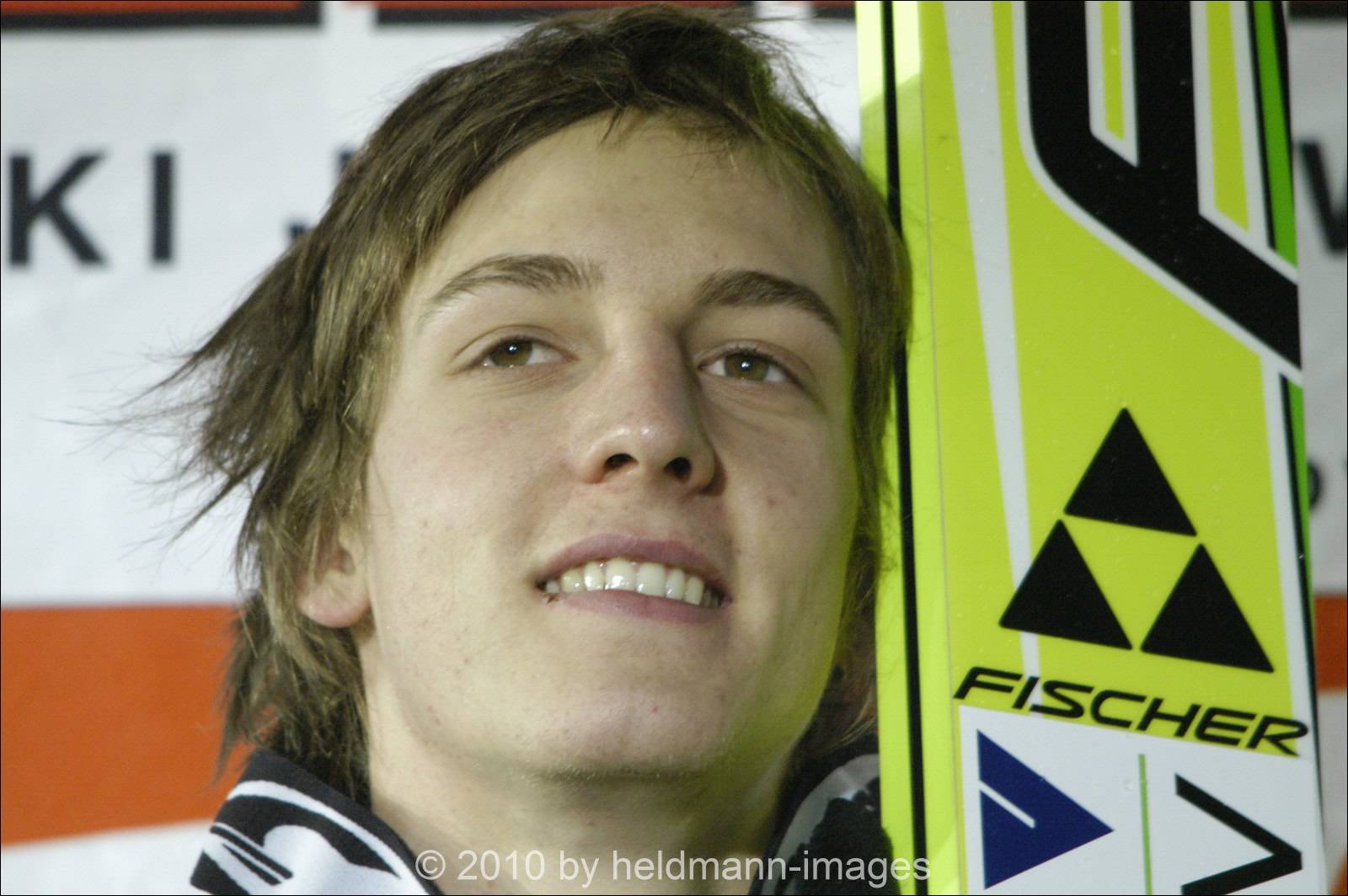In this image, a man with light brown hair and light brown eyes takes center stage, his head slightly tilted to the right and eyes gazing upward to the left. The close-up captures him smiling faintly, revealing the top row of his teeth. He sports a black and white outfit, and the top of his head nearly touches the top of the frame. The background blends into the scene but provides context clues to the setting: there is a blurry poster or signage with indistinguishable content, possibly indicating a sporting event, and a board off to the right prominently displays the name "Fisher." Additional colors in the background include lime green, dark blue, gray, red-orange, yellow, and black, enhancing the energetic atmosphere. A copyright notice at the bottom of the image states "2010 by Heldman Images."